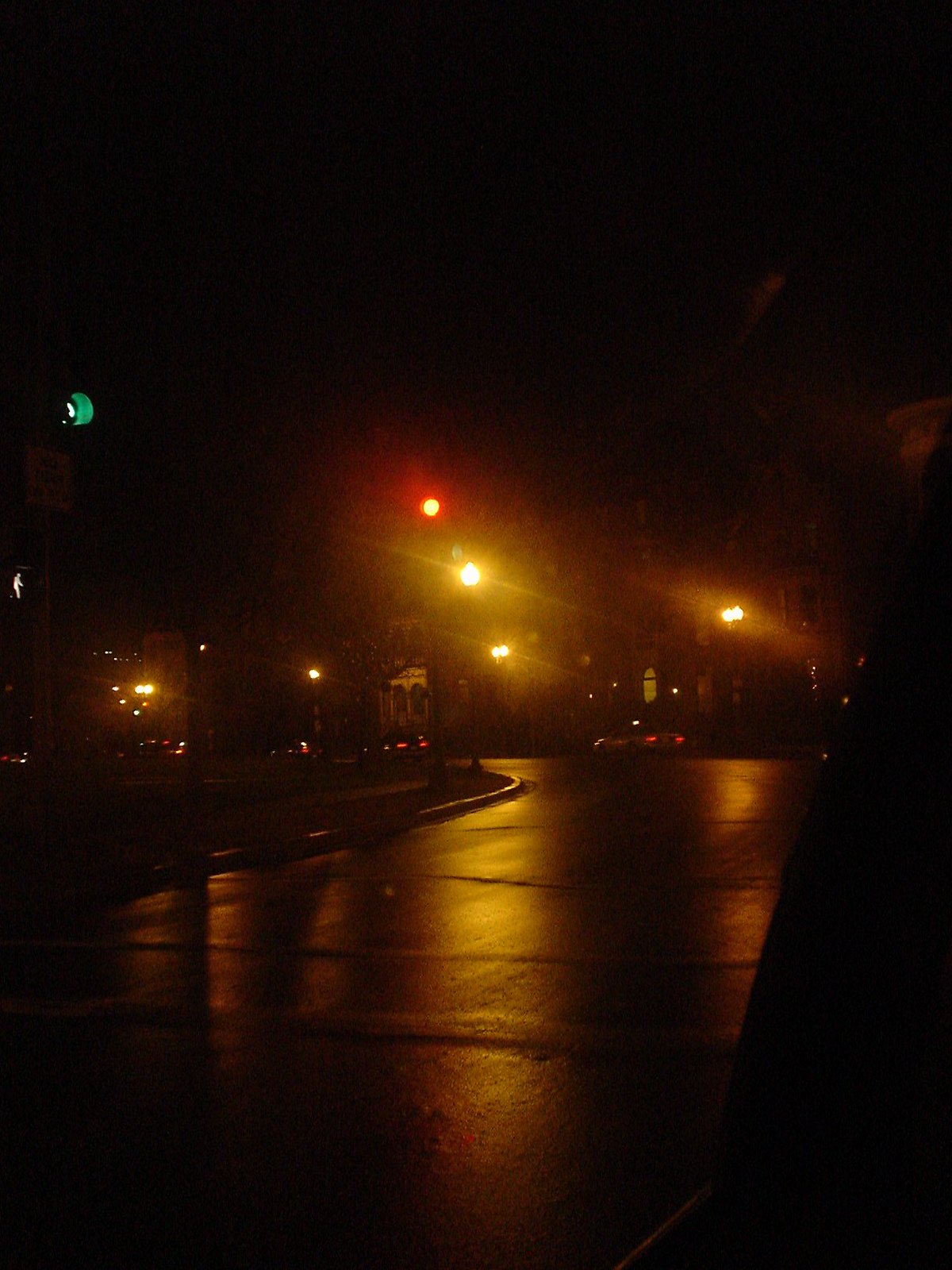Captured on a nighttime stroll through a bustling business district, this photograph reveals a vibrant streetscape under the glow of various streetlights. On the left, a green light hangs prominently, accompanied by a walk sign indicating it's safe for pedestrians to cross. Ahead in the distance, a red light casts a cautionary glow. The glare from multiple streetlights creates a luminous haze over the scene. The road curves sharply to the left, suggesting the intricate layout of the area. On the right, a series of buildings line the street, reminiscent of structures found in smaller towns. A white car is parked on the right, followed by three other vehicles navigating the curve in the opposite lane. The photo encapsulates the dynamic interplay of light and architecture in an active urban setting.